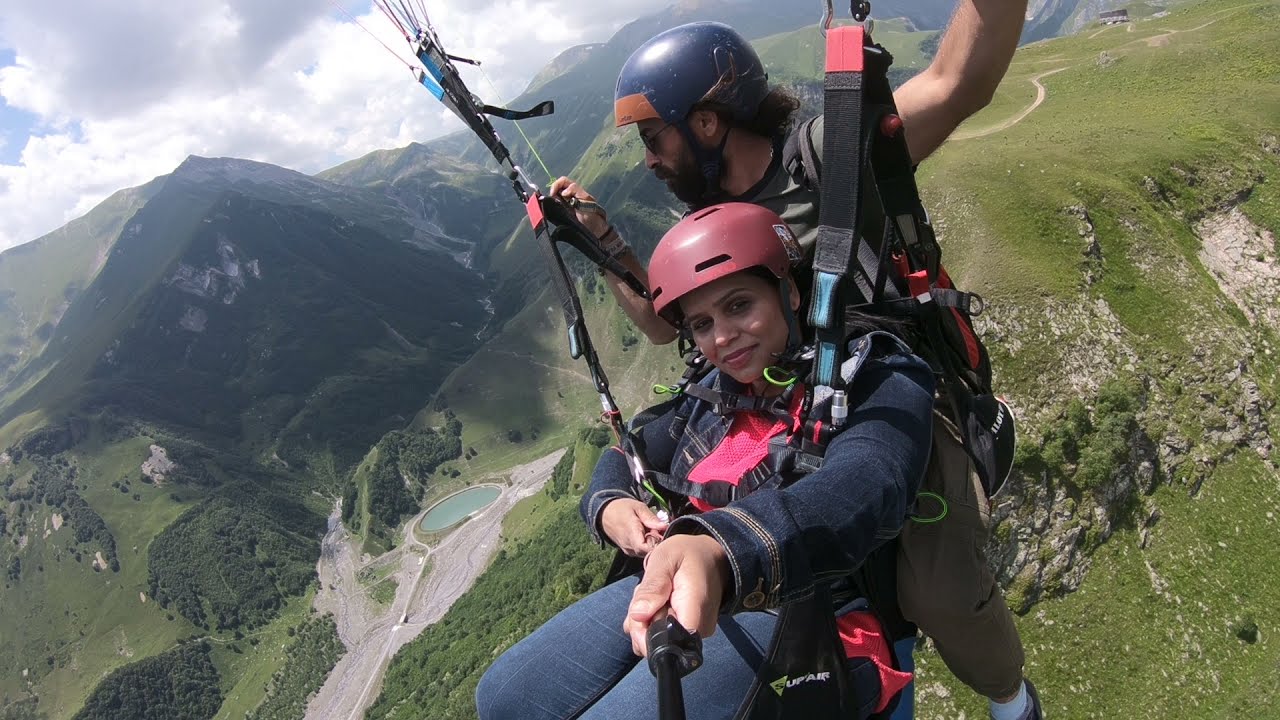In this adventurous and exhilarating full-color photograph, captured outdoors on a partly sunny, cloudy day, two people are tandem skydiving high above a lush, mountainous landscape. Below them, the terrain is dotted with green foliage, rocky outcrops, and a distinct, round man-made body of water. The woman in the foreground, dressed in blue jeans, a pink shirt, and a denim jacket, is wearing a burgundy helmet and holding a selfie stick, capturing the thrilling moment. Behind her, the man, sporting a full beard, sunglasses, blue and orange helmet, and green cargo pants, is managing the parachute. His arms appear to be controlling their descent, and while he looks off to the side, she gazes directly into the camera with a relaxed expression, suggesting she is enjoying the experience. The mountainous backdrop and expansive view of trails, roads, and greenery contribute to the beauty and excitement of the scene.